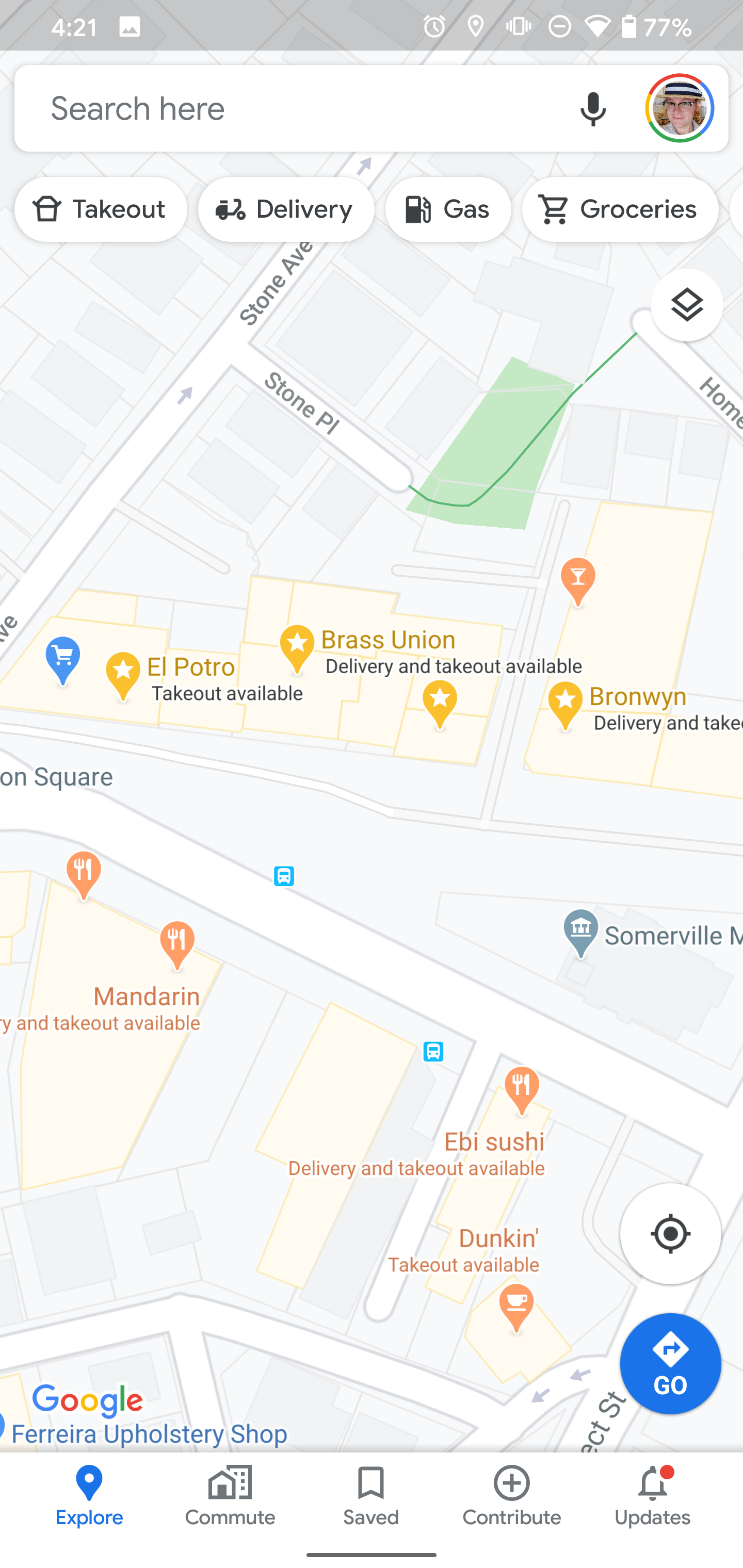This image is a screenshot from Google Maps, featuring various interface elements and a section of a mapped area with highlighted points of interest.

At the top of the image, there is a long gray bar displaying the current time (4:21) on the left and a battery icon showing 77% on the right. Below this bar, a search box is centrally positioned with the text "Search here" inside it, and to its right, there is a circular avatar image of a person’s face. Underneath the search box, there are elongated circular buttons labeled as "Takeout," "Delivery," "Gas," and "Groceries."

The main part of the image shows a detailed map. Prominent streets on the map include Stone Point and Stone Avenue. There are several yellow markers indicating locations such as:
- El Porto, which offers takeout.
- Brass Union, which provides both delivery and takeout services.

A distinctive white diagonal line, representing a roadway, cuts across the map. Below this line, an orange marker points to "Mandarin," and further markers indicate:
- EBI Sushi, marked with an orange fork and knife icon.
- Dunkin, which also offers takeout and is marked similarly with an orange fork and knife icon.

Towards the bottom right corner, there is a blue circle with the word "GO" inside it.

At the very bottom of the image, there are four clickable options labeled "Explore," "Save," "Contribute," and "Updates." Above the "Updates" option, there is a red dot placed above a bell icon, signifying a notification.